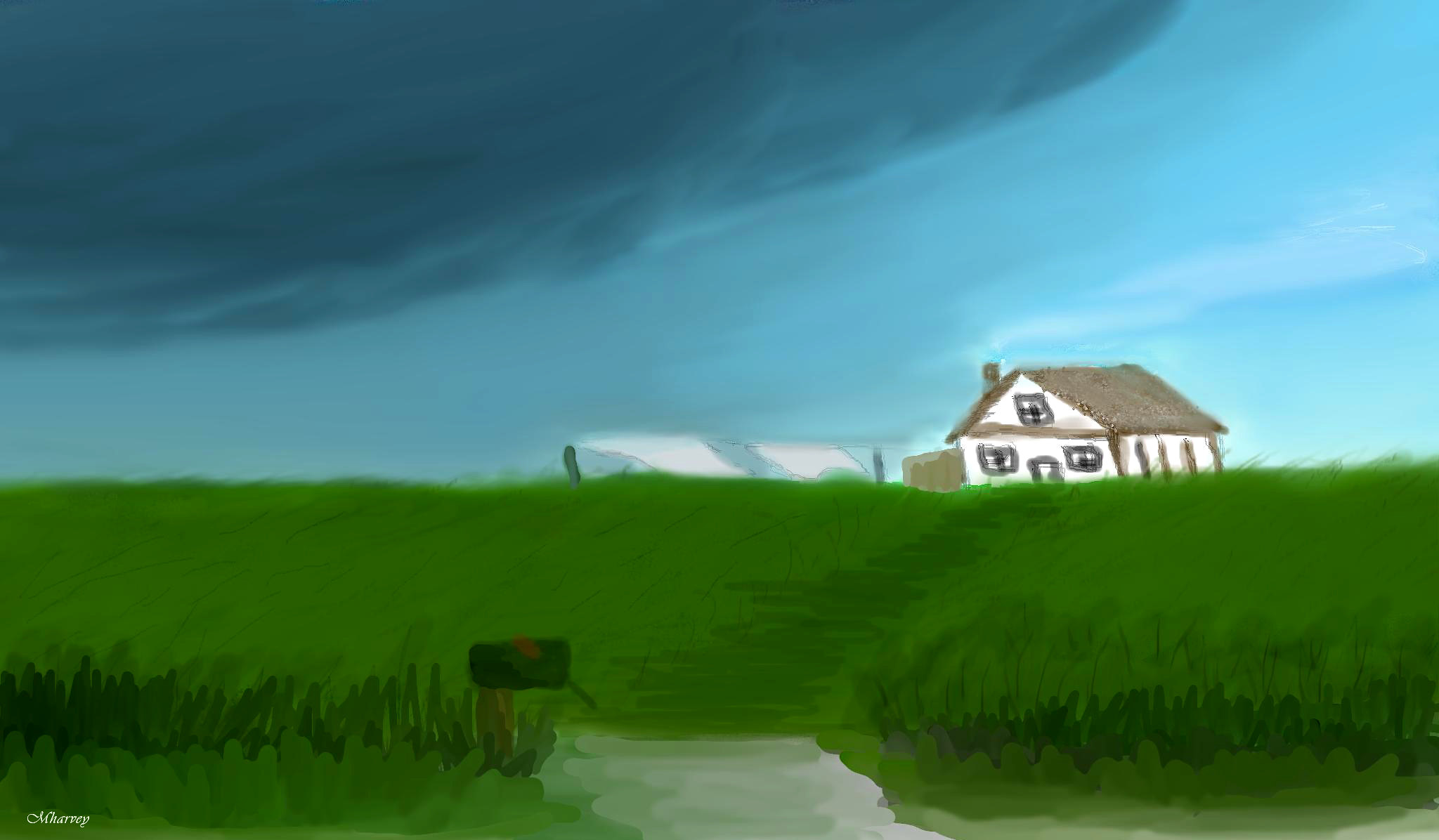This watercolor painting captures a scene reminiscent of the opening shot of The Wizard of Oz. It depicts a solitary white farmhouse situated in the middle of an expansive, open landscape, with a dramatic storm approaching from the distance. The sky above is divided between patches of serene blue and ominous gray clouds, signaling the impending arrival of the storm. The farmhouse, simple yet charming, features a few windows, a doorway, and is surrounded by lush green grass. A clothesline with laundry flutters in the wind, adding a touch of daily life to the scene. The painting is completed with a dirt road that leads away from the farmhouse, inviting viewers to imagine the unfolding story of the rural homestead bracing for nature's fury.